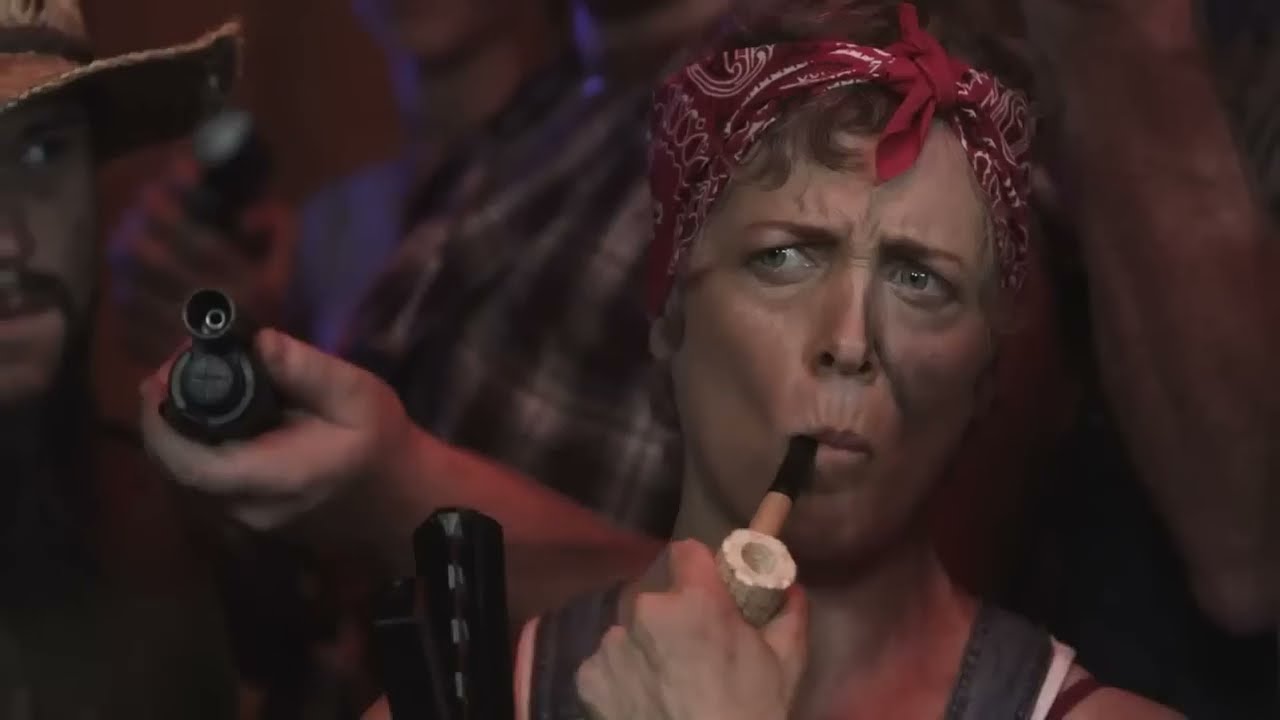In this apparent screen grab from an intense action movie scene, a middle-aged woman with a weathered face, marked by wrinkles around her mouth and forehead and shadowed cheeks, is centrally framed. She has a red paisley bandana tied around her head and is smoking from a corncob pipe. Her expression is a mix of caution and concern, giving the impression that she's deeply pondering or weighing a critical decision. Her attire includes a tank top, and her face appears dirty, heightening the gritty atmosphere of the scene. Directly behind her, a man dressed in a black and white flannel plaid shirt is aiming a shotgun towards the camera, adding a sense of imminent danger. To his side, another man with a beard, wearing a cowboy hat, is partially visible, looking off to the side. The blurred background accentuates the sharp focus on the tense expressions and the shotgun, suggesting a pivotal moment in the storyline.